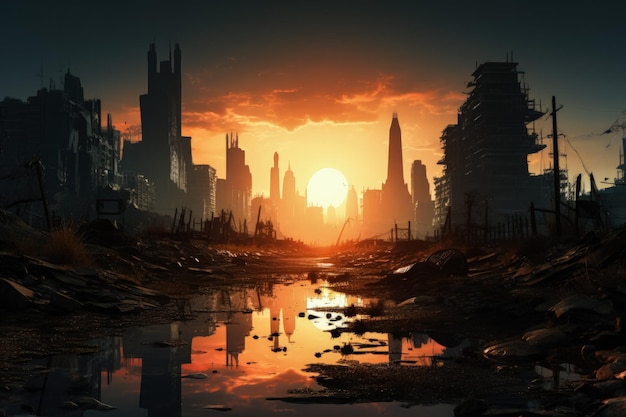This computer-generated image depicts a dystopian cityscape at either sunrise or sunset, casting an eerie atmosphere over the scene. Dominating the center of the image is a large, golden-orange sun, partially obscured by clouds that transition from golden-orange near the sun to dark and stormy further up. The sun's light reflects off a narrow, swampy river running down the middle of the image, surrounded by debris, such as fallen building materials, tires, and damaged fences. On either side of the river are abandoned and crumbling buildings, starkly shadowed and appearing desolate and unmaintained. The background features distant, slightly more intact skyscrapers. The entire scene is enveloped in a golden-yellow haze, contributing to the overall sense of ruin and decay that defines this dystopian landscape.